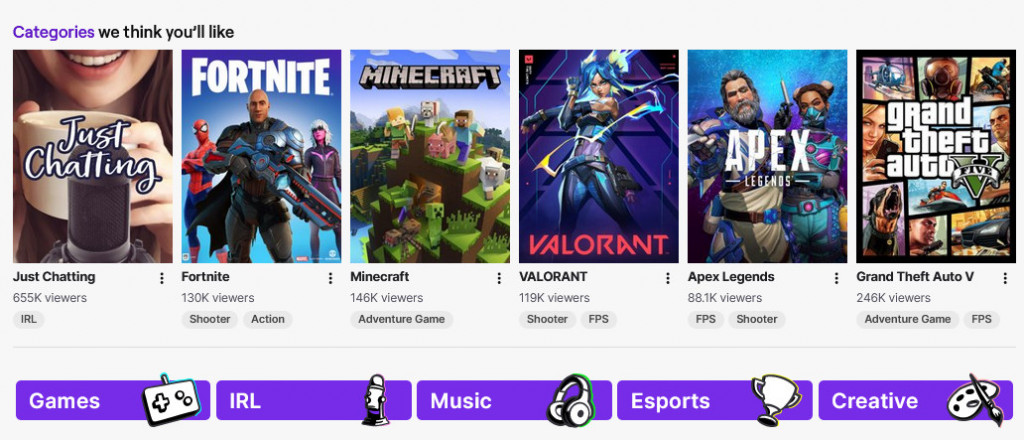A horizontal screenshot of the Twitch website showcases several tabs and categories prominently. At the top left corner, purple text reads "Categories," while adjacent black text states "We Think You'll Like." Below these headings are six distinct streaming categories:

1. The first category, "Just Chatting," features an image of a woman sipping from a white mug with a microphone in front of her. The category name appears twice: once centrally in white text with a black border, and again in black text underneath.
2. Next, the "Fortnite" category portrays three distinctive characters with the game title "Fortnite" in bold white text at the top.
3. The "Minecraft" category displays iconic characters such as Steve, Alex, a wolf, pigs, sheep, and creepers atop a grassy hill. The title "Minecraft" is visible at both the top and bottom of the image.
4. Following this, the "Valorant" category showcases a central figure of a woman with bright blue hair.
5. The "Apex Legends" category features two characters positioned centrally— a man on the left and a woman on the right— with the game title "Apex Legends" in white text in the center.
6. Lastly, the "Grand Theft Auto V" category consists of multiple panels depicting various characters in a cartoonish style. The title "Grand Theft Auto V," with the numeral "V" in Roman format, is centered in white text.

At the bottom of the screenshot, five purple tabs are labeled from left to right: "Games," "IRL," "Music," "Esports," and "Creative," each in white text.